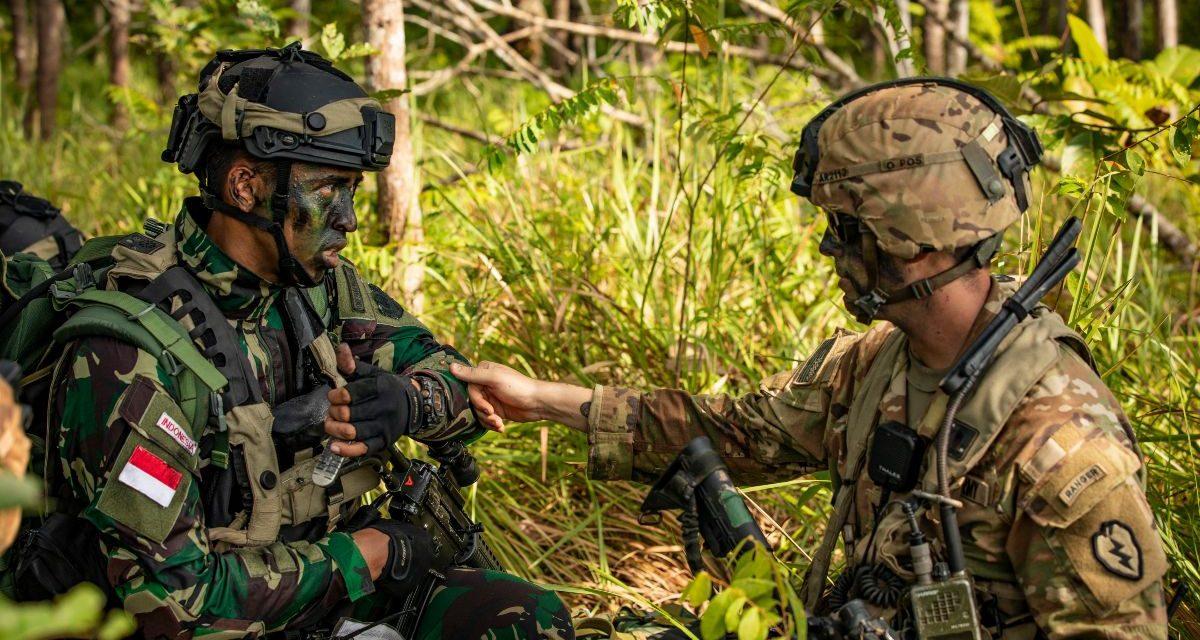In the rectangular photograph, which is lush with green vegetation and tall grass, two soldiers from different nations are engaged in a conversation while sitting in a grassy, forested area. The soldier on the left, wearing dark brown, green, and tan camouflage, has a black helmet with a tan strap around it and a red-and-white flag on his sleeve, indicating his Indonesian affiliation. He is equipped with black fingerless gloves, a green backpack, a tan-colored chest harness, and a black rifle. His face is painted in black and green camouflage. The soldier on the right is dressed in lighter brown, tan, and green camouflage. On his sleeve, he wears an American flag and a patch featuring a lightning bolt and the word "Ranger." This soldier is also equipped with numerous pieces of equipment, including sunglasses, a tactical helmet, and a walkie-talkie. He is seen reaching out with his right hand and gripping the sleeve of the soldier on the left. The backdrop of the image features tall trees, branches, and leaves, providing a dense, forested environment. Additionally, there appears to be another individual partially visible on the right side of the frame.